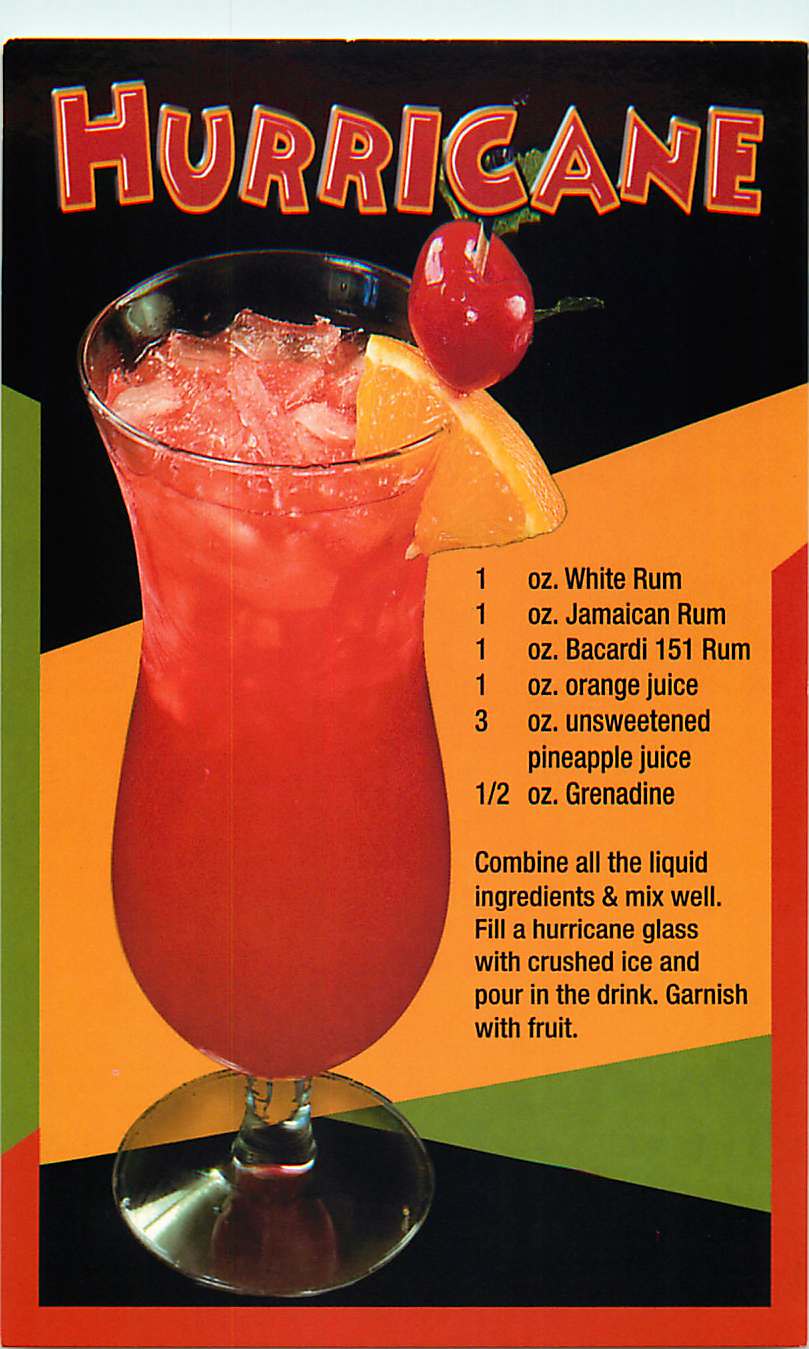This vibrant ad showcases a hurricane drink recipe, prominently featuring a tall, shapely glass filled with the vibrant red drink, topped with a toothpicked orange wedge and cherry garnish. The background bursts with blocks of black, green, yellow, and red colors, creating an energetic and engaging visual. At the top, the word "Hurricane" stands out in bold, fun red lettering with an orange outline. Detailed instructions in black text outline the recipe: 1 ounce white rum, 1 ounce Jamaican rum, 1 ounce Bacardi 151 rum, 1 ounce orange juice, 3 ounces unsweetened pineapple juice, and a half-ounce of grenadine. It directs to combine all liquid ingredients, mix well, fill a hurricane glass with crushed ice, and garnish with fruit. The layout is meticulously crafted, with the drink image front and center, exuding a lively, celebratory vibe.